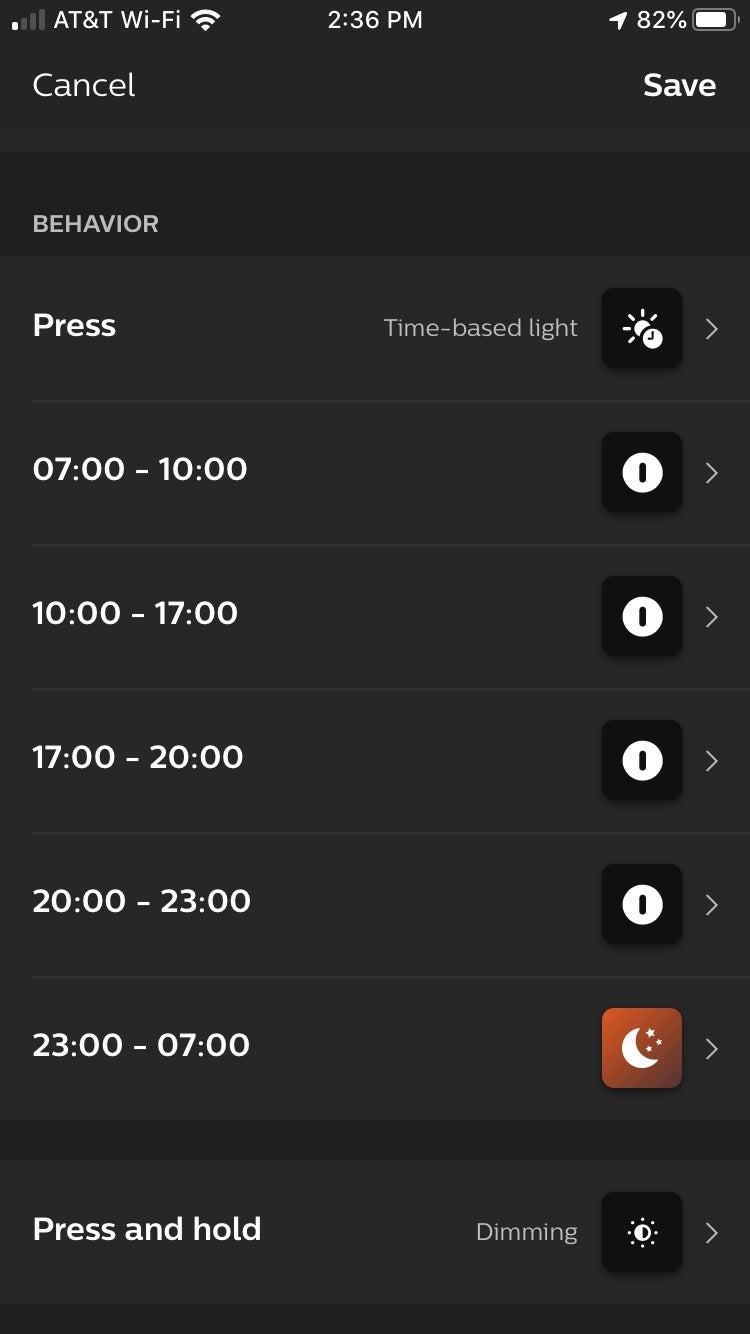In the image, the top-left corner displays one bar of AT&T Wi-Fi signal alongside the current time of 2:36 p.m. The top-right corner shows a kitchen service notification at 82%, with options such as 'Cancel,' 'Save,' and 'Press,' indicating a time-based schedule. The notification is gray and includes a timetable that starts from 1 to 7, then from 10 to 17, followed by 17 to 20, and finally from 20 to 23 hours. Below this, numbers seem continuous, extending from 23 to 7. There is also a red square icon accompanied by a half moon symbol, suggesting nighttime mode or a similar feature. On the bottom-left side, there is an instruction to 'Press and Hold,' with the text dimming gradually. The bottom-right corner shows a detailed icon featuring 7 rays, suggesting different sections or options.